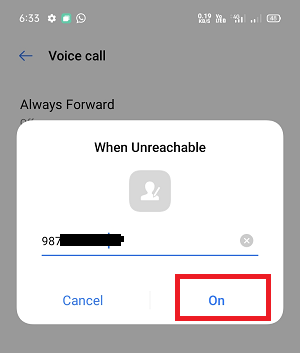The image displays a user interface with multiple visual elements layered on a dark gray square background, which has the number "633" displayed prominently. 

At the top of the gray square, there is a smaller white square overlay. This white square contains various icons: 
- A settings icon.
- A folder icon.
- A speech bubble icon that encases a phone symbol.

Below these icons is a blue arrow pointing to the left, next to which the words "voice call" appear in small black letters. Subsequently, the phrase "always forward" is written in regular black font.

In the center of the composition, another white square sits on the gray background. This white square displays the text "when unreachable" in black letters. Below this, there is a smaller gray square with a white icon of a person inside it.

A phone number, obscured by a marking resembling the shape of a AA battery, appears beneath this smaller gray square. Next to this obscured number is a blue line. Adjacent to the blue line, a gray circle with a white "X" is positioned.

Underneath the blue line, the word "cancel" is written in blue text. At the bottom of the image, there is a red rectangle containing the word "ON" in blue letters.